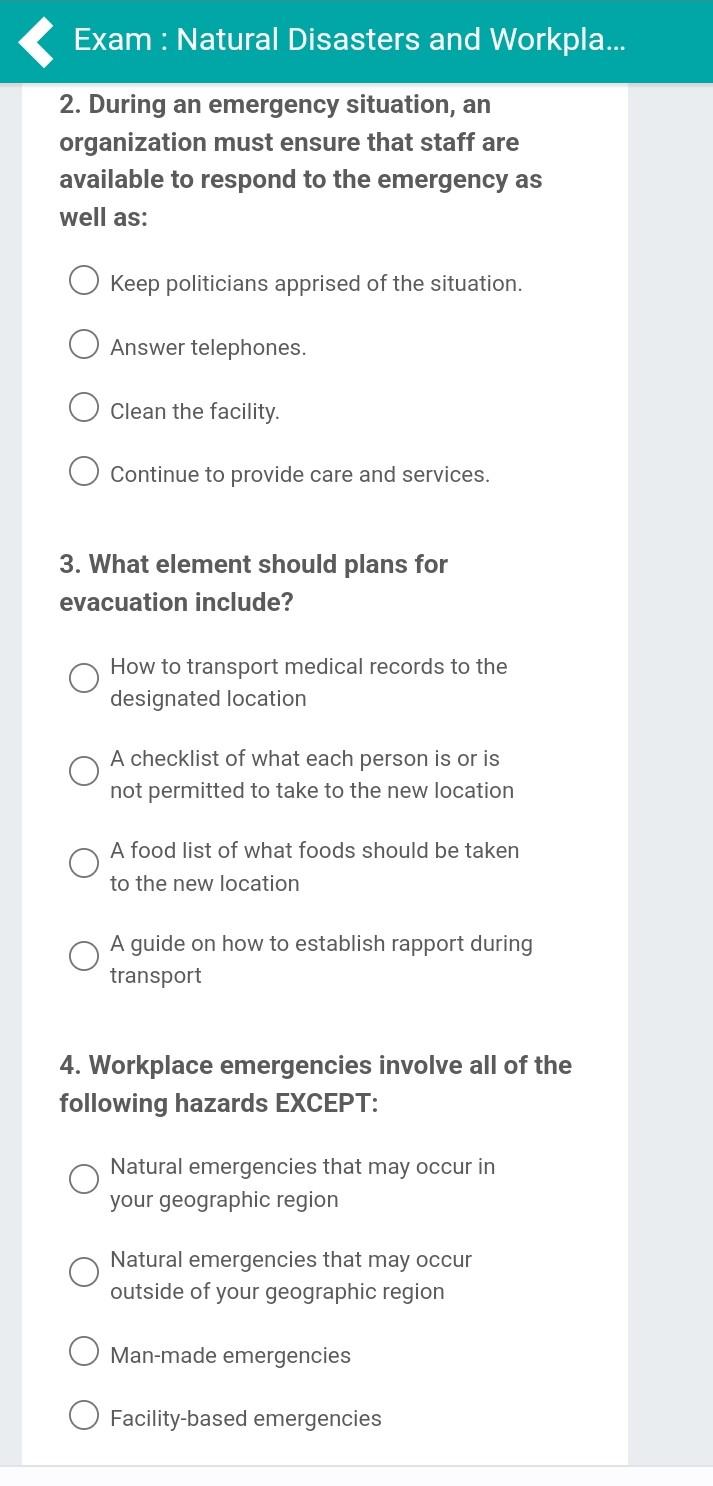In this image, we observe a screenshot of a web page dedicated to an examination on natural disasters and emergency preparedness. The top of the page features a green header or banner with bold, white text. Prominently displayed within the banner is a large arrow pointing to the left, and to the right of this arrow is the word "Exam." 

Beneath the header, against a white background, is Question 2 of the exam. The question reads: "During an emergency situation, an organization must ensure that staff are available to respond to the emergency as well as..." This is followed by four multiple-choice answers, each with a small circle to the left for selection. The options are:
1. Keep politicians apprised of the situation.
2. Answer telephones.
3. Clean the facility.
4. Continue to provide care and services.

Following this is Question 3, asking: "What elements should plans for evacuation include?" Again, four options are provided:
1. How to transport medical records to the designated location.
2. A checklist of what each person is or is not permitted to take to the new location.
3. A food list of what food should be taken to the new location.
4. A guide on how to establish rapport during transport.

The web page thus offers a structured set of questions and answer choices designed to test knowledge on emergency response and evacuation procedures.